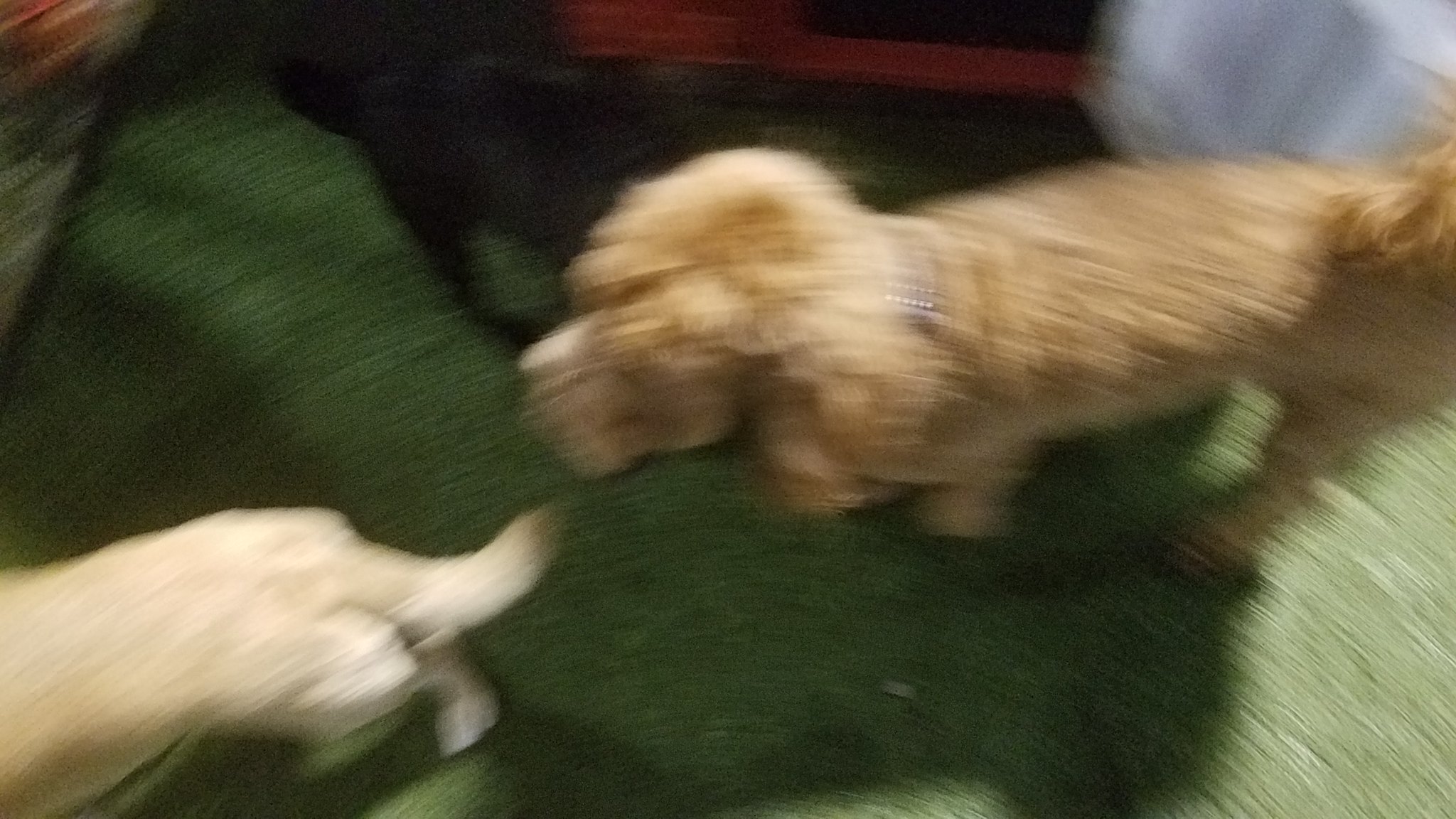The image captures a top-down view of two dogs standing on a green surface, likely astroturf or a carpet, given the out-of-focus and blurry nature of the photograph. The dog on the right, predominantly featured, has a golden, blindish-brown coat with long, floppy, curly ears, and is wearing a collar. This dog resembles a spaniel and appears to be motionless. To the left of this dog is another dog, whose back half and tail are visible. This smaller dog has a lighter brown or white coat with distinct white legs and a white-tipped tail. Behind the dogs, a red table or structure is faintly discernible through the blur. Overall, the scene is somewhat indistinct due to the lack of focus and motion blur, but it evokes a sense of a casual moment captured outdoors on a synthetic green surface.